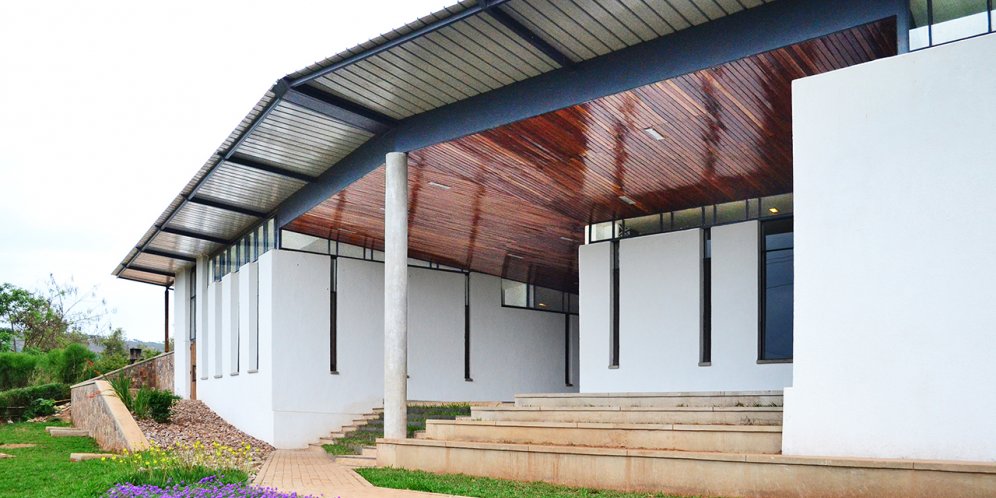The photograph captures the outside of a newly-constructed building on a cloudy day, under an overcast sky that appears white. The building's façade is painted white, with plenty of windows ensuring abundant indoor sunlight. The entryway is comprised of a light brown paved walkway flanked by lush green grass sprinkled with purple and yellow flowers. A set of unstained, light wooden steps leads up to a porch area, which is supported by a large, round column and features a roof with blue and light tan elements. The overhang is detailed with dark blue crossbeams and dark wooden slats, adding a touch of elegance to the structure. On the left, there is a retaining wall with rocks and a couple of bushes, complementing the manicured front yard. The porch ceiling inside is made of dark wood, contrasting the building's overall light tones.